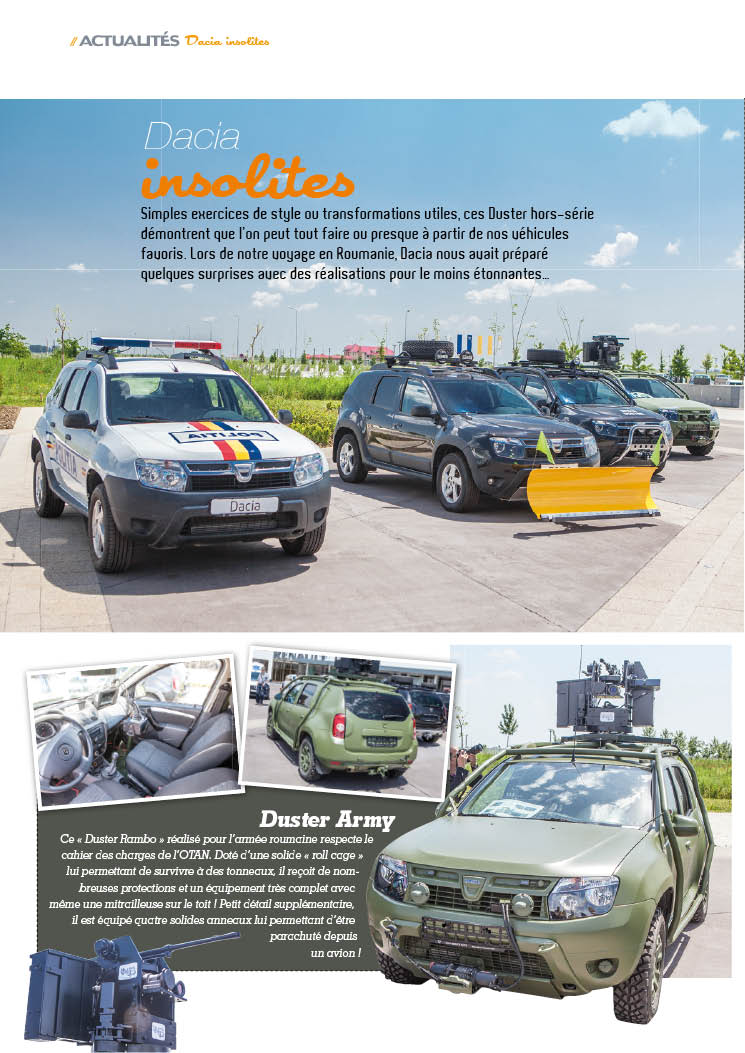The image appears to be an advertisement composed of two sections, both featuring cars. The top section displays a group of off-road vehicles commonly seen in Europe. There are emergency lights on top of a few, including one that has a yellow snow plow with green flags and another that has police markings. The text in the top section, which is in French, reads "Dacia Insolites." One of the vehicles even has a bulldozer attachment in front. The bottom section features a military green off-road vehicle, labeled "Duster Army," which is equipped with what looks to be a weapon turret on the roof. This vehicle is depicted from multiple angles, including its gray interior. All vehicles are stationary and lined in rows against a backdrop of blue skies on a sunny day. The shared theme across both parts heavily emphasizes off-road capabilities and special modifications for emergency and military applications.